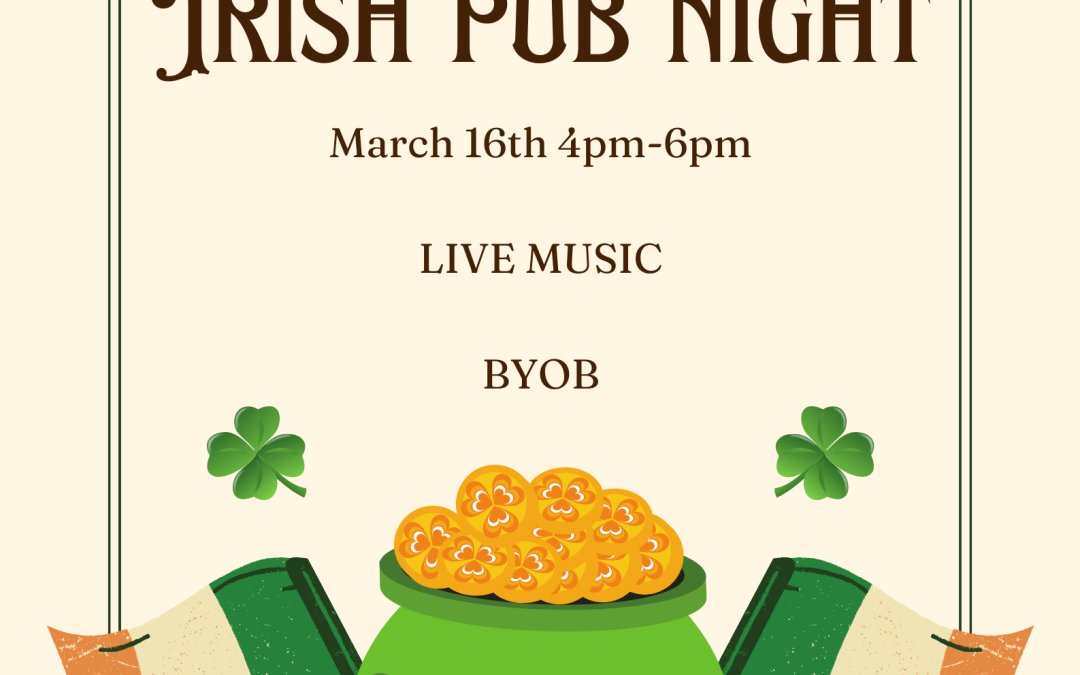The image is an advertisement for an Irish Pub Night, prominently featuring the event details at the top, albeit partially cropped. The text reads "Irish Pub Night" in brown, followed by "March 16th, 4 p.m. to 6 p.m.," and underneath that, "Live Music" and "BYOB," all in a similar brown, all-caps font. The background is white, and the design is simple, with a clip-art style. At the bottom, a green pot filled with cartoon gold coins adorned with three-leaf clovers takes center stage. Flanking the pot are partially visible Irish flags and additional shamrock symbols, enhancing the St. Patrick's Day theme. The overall appearance is elementary and lacks professional design elements.